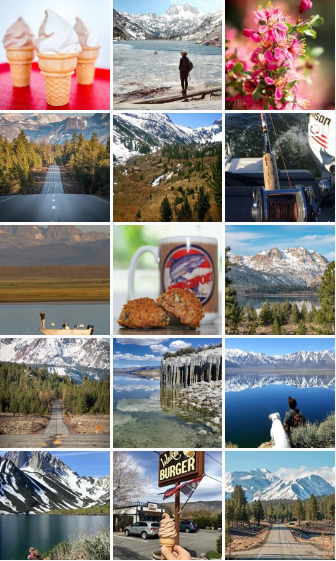The image is a neatly arranged 3x5 grid of 15 uniform square photos, all separated by crisp white lines and set against a white background. Each photo is evenly spaced, creating a clean and organized layout. Here's a detailed breakdown of the images from top left to bottom right:

1. A vibrant red plate holding a beautifully swirled ice cream cone.
2. A person gazing at majestic glaciers, captured mid-contemplation.
3. A cluster of delicate pink flowers, blooming vibrantly.
4. An angler poised with a fishing rod, set against a serene outdoor backdrop.
5. A panoramic view of jagged mountains and icy glaciers.
6. A quiet country road flanked by mountains and dense forest.
7. A scenic shot of someone riding a boat, framed by towering mountains in the background.
8. A mouthwatering plate of crab cakes accompanied by a seafood cocktail.
9. Forest-covered mountains rising majestically in the distance.
10. A pair of playful dogs posing in front of a tranquil lake, with mountains looming behind.
11. Icicles delicately dripping into a serene lake.
12. Another perspective of a country road, this time more of the mountain base is visible.
13. A picturesque lake edged by a rugged mountain.
14. An ice cream cone poised enticingly in the foreground of a classic hamburger diner.
15. A country road with a sweeping view of an entire mountain range.

Each photo captures a unique and beautiful aspect of nature and daily life, forming a visually appealing and cohesive collection.